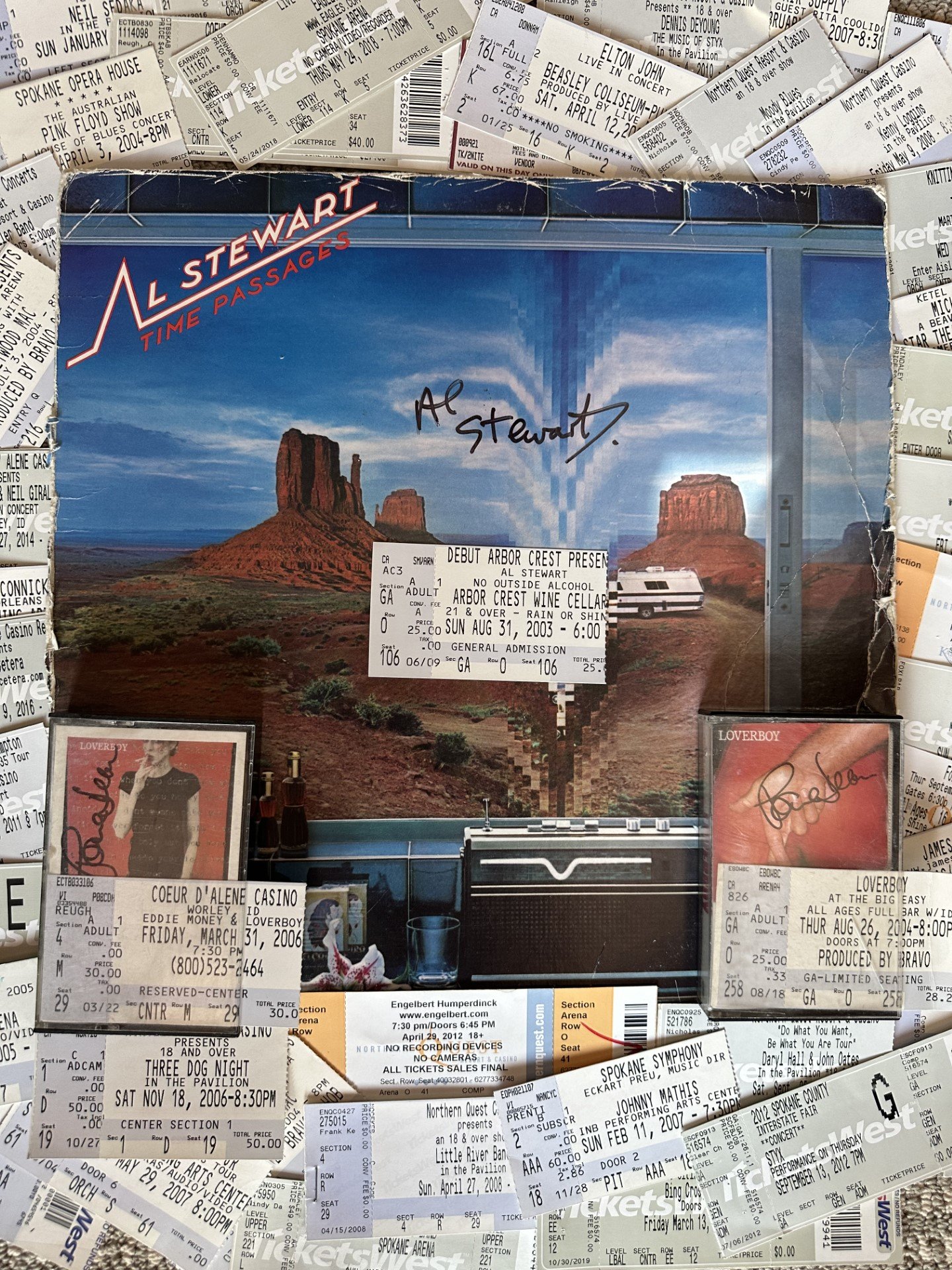This image is a meticulously crafted collage showcasing a diverse collection of concert tickets from various venues and events. The background is densely packed with an array of Ticketmaster stubs from notable performances, including Elton John, the Spokane Opera House with Pink Floyd, and the Spokane Symphony featuring Johnny Mathis. At the center, an Al Stewart "Time Passages" record is prominently displayed, featuring an American desert landscape with what appears to be an RV, possibly in the Arizona or Utah desert, under a blue sky. The record is autographed by Stewart himself. Surrounding the record are two autographed cassette tapes and additional memorabilia, including a debut Arbor Crest ticket and a Coeur d'Alene Casino ticket. Among these, a Loverboy CD with a striking red label and cover stands out. This collage captures not only the variety of musical acts but also the personal significance of the collection, as noted by the signatures and carefully arranged items, creating a layered snapshot of concert history and cherished memories.